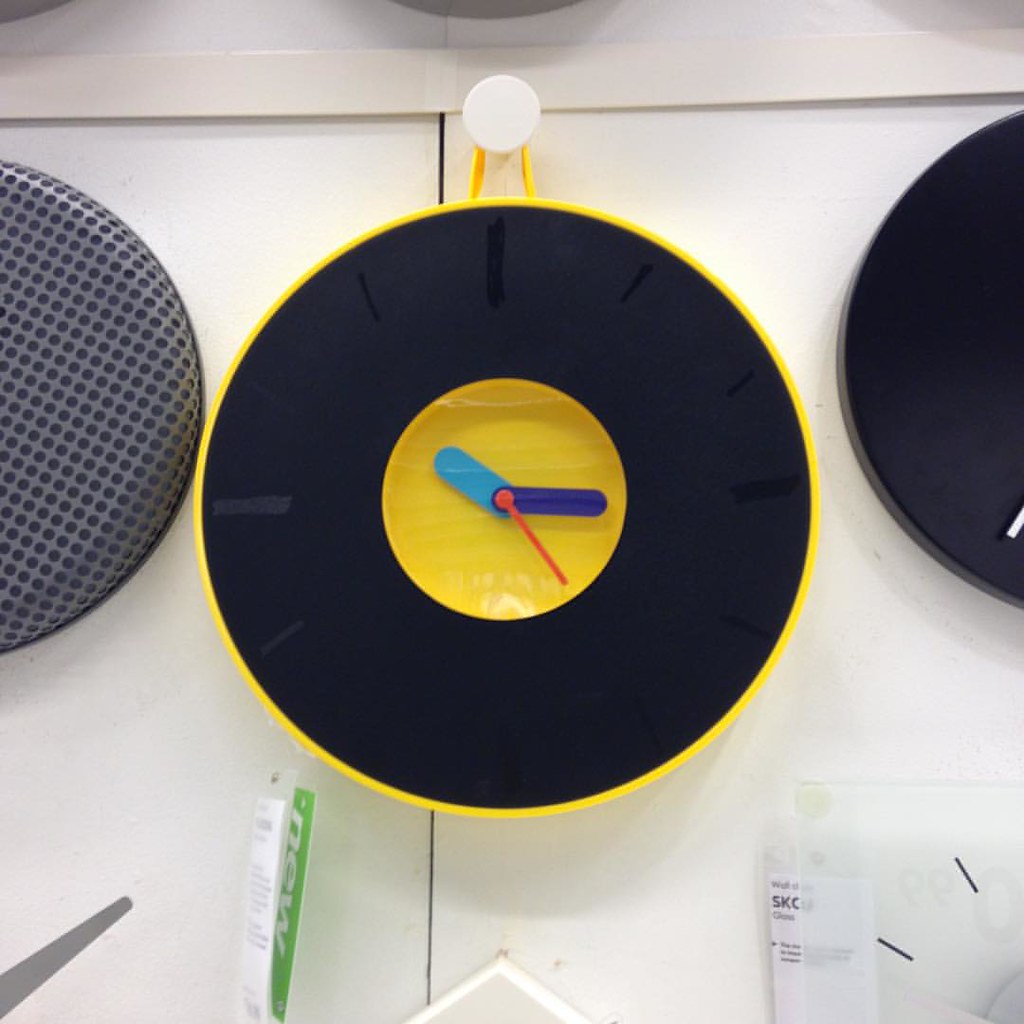The photograph features a uniquely designed clock resembling the shape of a donut. The main circular body of the clock is black, encircled by a thin yellow border. Dominating the center, reminiscent of a donut hole, are the clock's hands: a light blue hand for hours, a purple hand for minutes, and a thin red hand for seconds. The hands indicate the time as 10:15 and 24 seconds. Instead of traditional numbers, the clock face is marked with 12 dashes representing each hour. The clock is set against a white background and appears to be hanging alongside two other clocks, of which only partial views are visible.